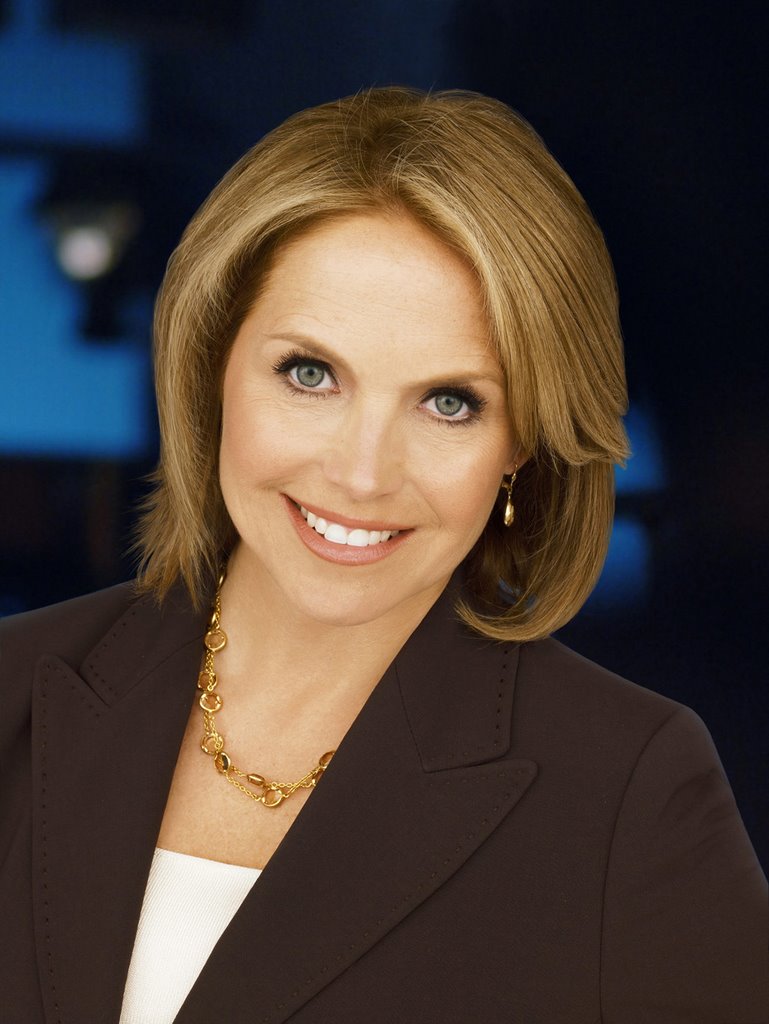This image features a younger Katie Couric, the famous journalist known for her work on NBC's "The Today Show." She has a cheerful smile, looking directly at the camera. Katie is dressed in a dark brown suit jacket over a white camisole. Accessorizing her outfit, she wears a gold necklace adorned with circular designs, and matching gold earrings. Her medium brown hair is straight and falls gracefully to her shoulders. Katie's eyes are highlighted with green makeup, adding a lively touch to her appearance. The background of the image is blurred, showcasing ambiguous shades of black and blue, with a hint of white on the left side that could be part of the setting or lighting.